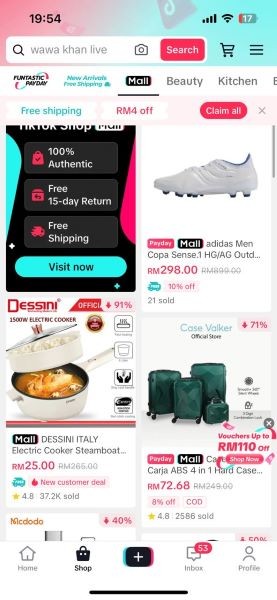The image depicts a non-American online auction or shopping website displayed on a smartphone screen. The phone's battery is at 17%. The search bar reads "wah-wah con live," indicating a potential marketplace or live auction feature. It appears that the user is browsing the mall section of the website, which prominently features offers such as "Free Shipping," "RM4 Off," "Claim All," "100% Authentic," "Free 15-Day Returns," and "Visit Now."

There are several featured items displayed:
- A pair of shoes priced at $298.
- A 1500-watt electric cooker, advertised with a 91% discount, though no specific price is mentioned.
- A hard case luggage set branded as "Carja ABS 401," priced at $72.

The currency used on the website is represented as "RM," which is unfamiliar in the context. Below these items, additional listings become obscured and are not clearly visible.

The bottom menu of the app includes navigation options labeled as "Home," "Shop," "Inbox," and "Profile." The overall layout and currency usage suggest that this is an international shopping platform.